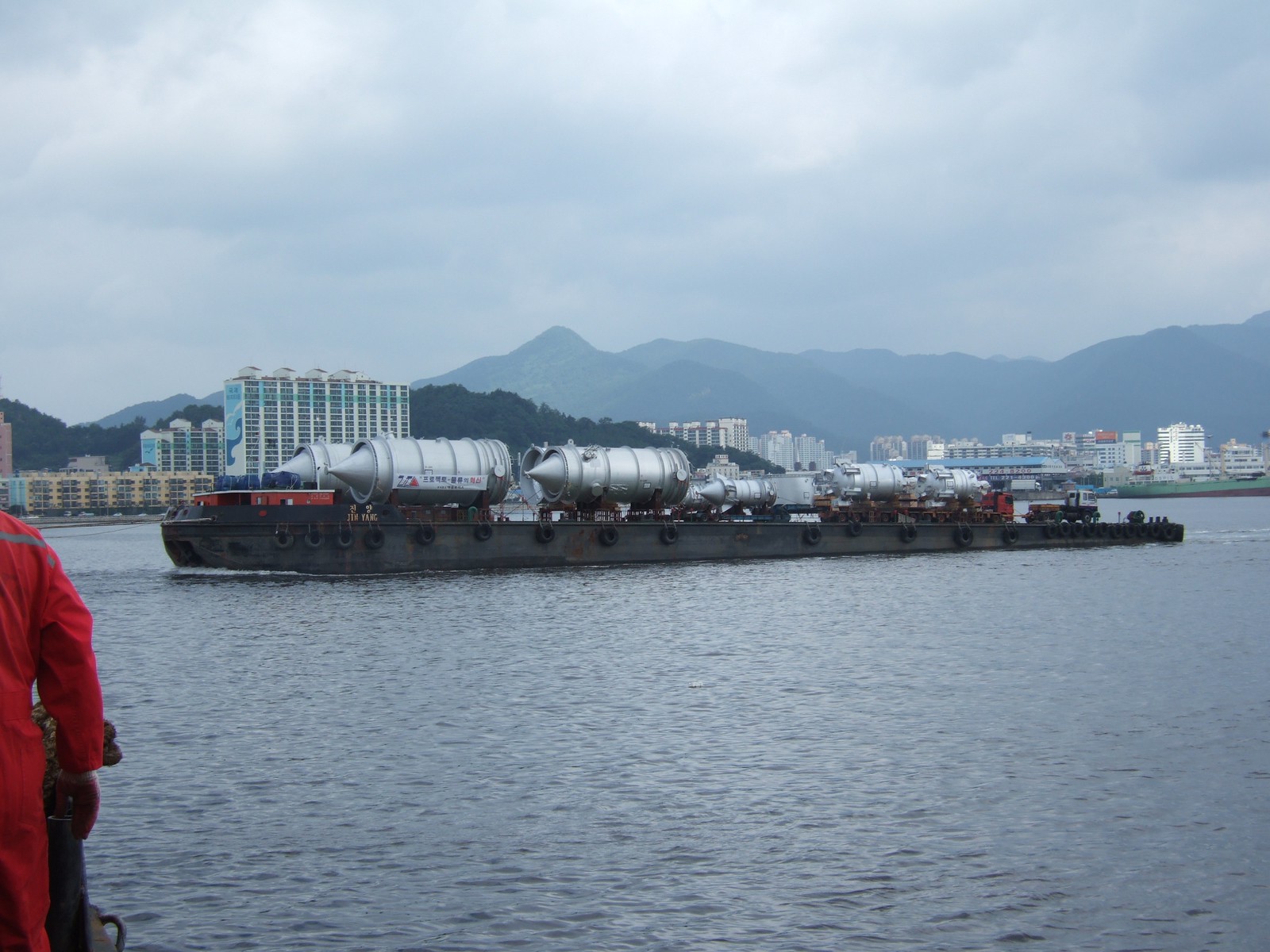The image depicts a large military-style ship navigating a river on an overcast day. The ship's hull is black on the bottom, transitioning to red towards the top, where the crew would be stationed. It is hauling several large, silver cylindrical objects that could be missiles or jet engines, notable for their pointed ends resembling cones or pyramids. The river is bordered by numerous large buildings, suggestively hotels, set against a backdrop of blue-gray mountains that resemble volcanoes, likely indicating a location such as Hawaii. In the lower left corner of the image, a person in a red jumpsuit with a reflective patch is seated in a small boat. The overall scene is marked by a predominance of gray tones, enhancing the somber, industrial atmosphere.